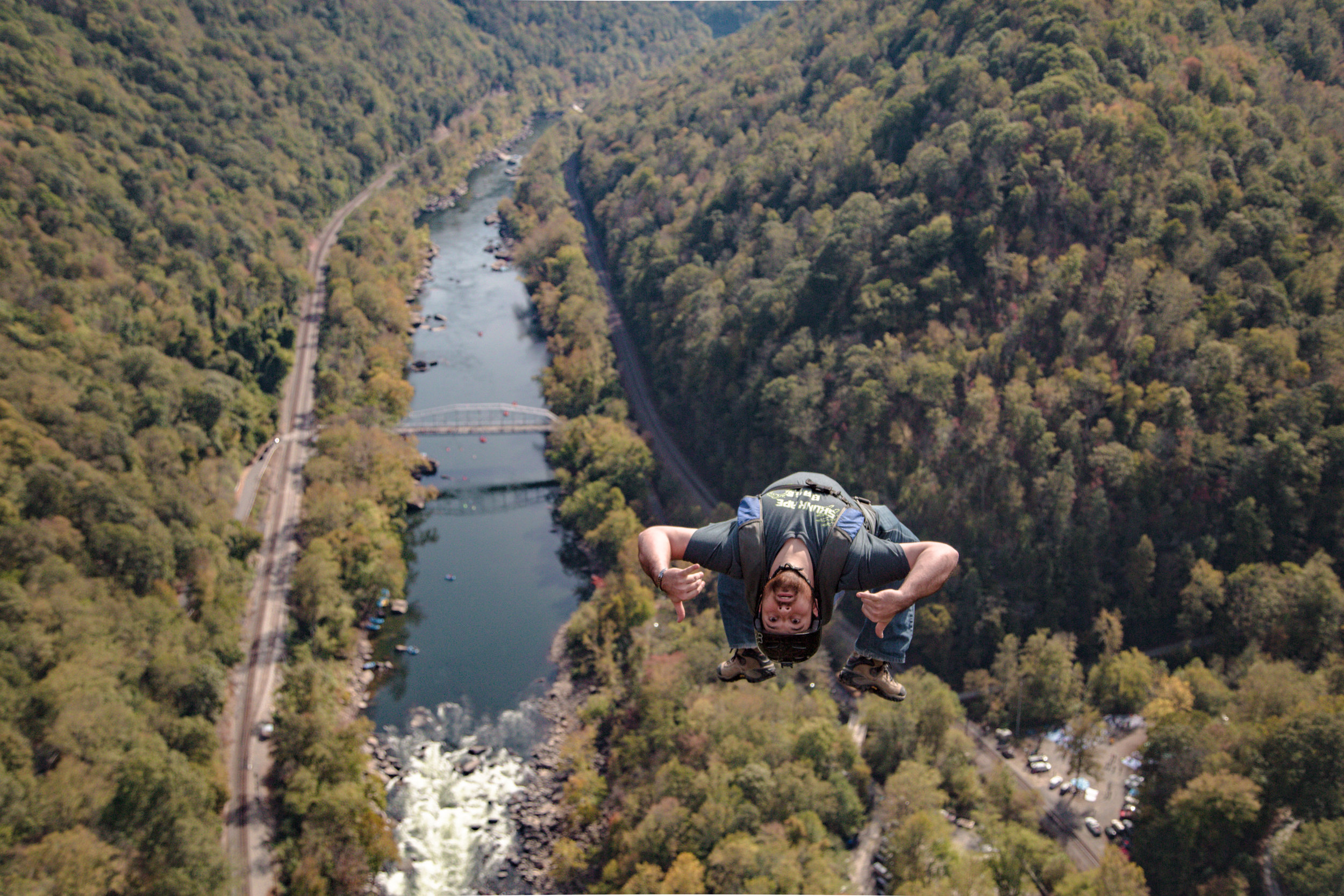This detailed aerial photograph captures a man mid-backflip in the vast sky. Facing the camera, his head is downwards, and his belly is up, with his hands extended upwards, conveying a sense of exhilaration. He is equipped with a helmet, jeans, boots, and a parachute backpack, clearly preparing for a skydive. The backdrop features a picturesque valley with a flowing river below, which is slightly to his left. The river, displaying shades of blackish-gray with foamy white water, is spanned by a bridge that connects roadways on either side. These roads traverse a landscape rich with lush green and autumn-hued trees, dotted with occasional pine trees. Mountains flank both sides of the valley, adding to the dramatic scenery. A parking lot with cars is also visible on the lower right, emphasizing the height from which this thrilling moment is captured.